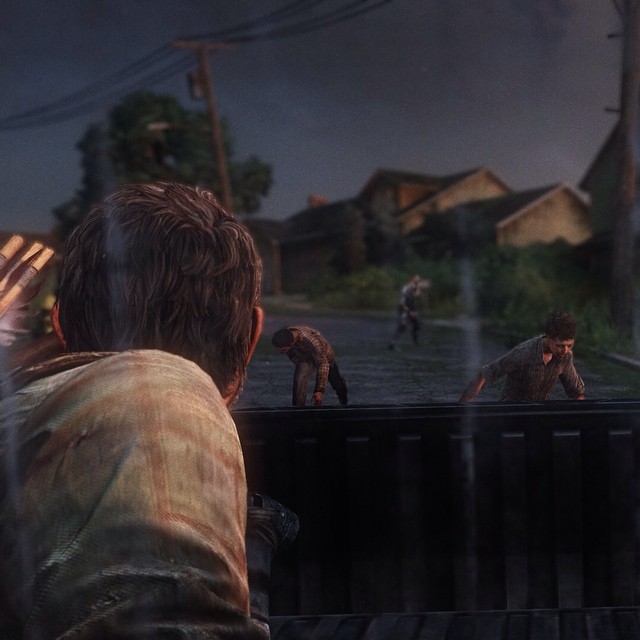The image appears to depict a computer-generated nighttime scene showcasing a dramatic and somber atmosphere. The sky is dark, setting the tone for the flooded street below. In the background, there is a split-level house with multiple floors and a garage door. The street is submerged in water, suggesting a severe flood.

In the foreground, three figures—likely two men and a boy—are wading through the water, walking towards the viewer. They all exhibit a hunched posture, possibly due to the difficulty of moving through the floodwaters. The foremost man has visible brown hair and a downcast face.

To the left of the scene, a telephone pole stands, partially submerged in the water. Nearby, the rear of a pickup truck is visible, with a man sitting on its left side. He is wearing a gray plaid shirt, has short brown hair, and white skin. Although initially it appears that his left hand is lifted, it is actually an unidentified tan object in the background. The man in the truck looks back at the trio wading through the water, adding to the narrative of concern or alertness in the scene.